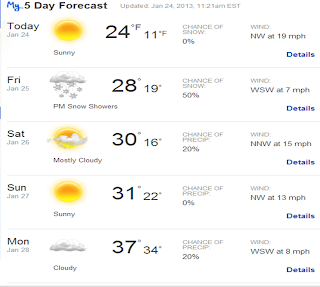Here is a detailed and cleaned-up caption based on the provided information:

---

The top section of the image displays a blue header reading "My Five-Day Forecast" with smaller gray text indicating the update time as "Updated January 24, 2013, 11:21 a.m. EST."

Below this, the weather forecast for the next five days is detailed as follows:

- **Thursday, January 24**: Sunny, with a high of 24°F and a low of 11°F. There is a 0% chance of snow, with winds coming from the northwest at 19 mph.
  
- **Friday, January 25**: Expect p.m. snow showers with a high of 28°F and a low of 19°F. The chance of snow is 50%, and winds will be from the west-southwest at 7 mph.
  
- **Saturday, January 26**: The day will be mostly cloudy, with temperatures reaching a high of 30°F and dropping to a low of 16°F. The chance of precipitation is 20%, and winds will be from the north-northwest at 15 mph.

- **Sunday, January 27**: Sunny, with a high of 31°F and a low of 22°F. There is no chance of precipitation, and winds will come from the northwest at 13 mph.